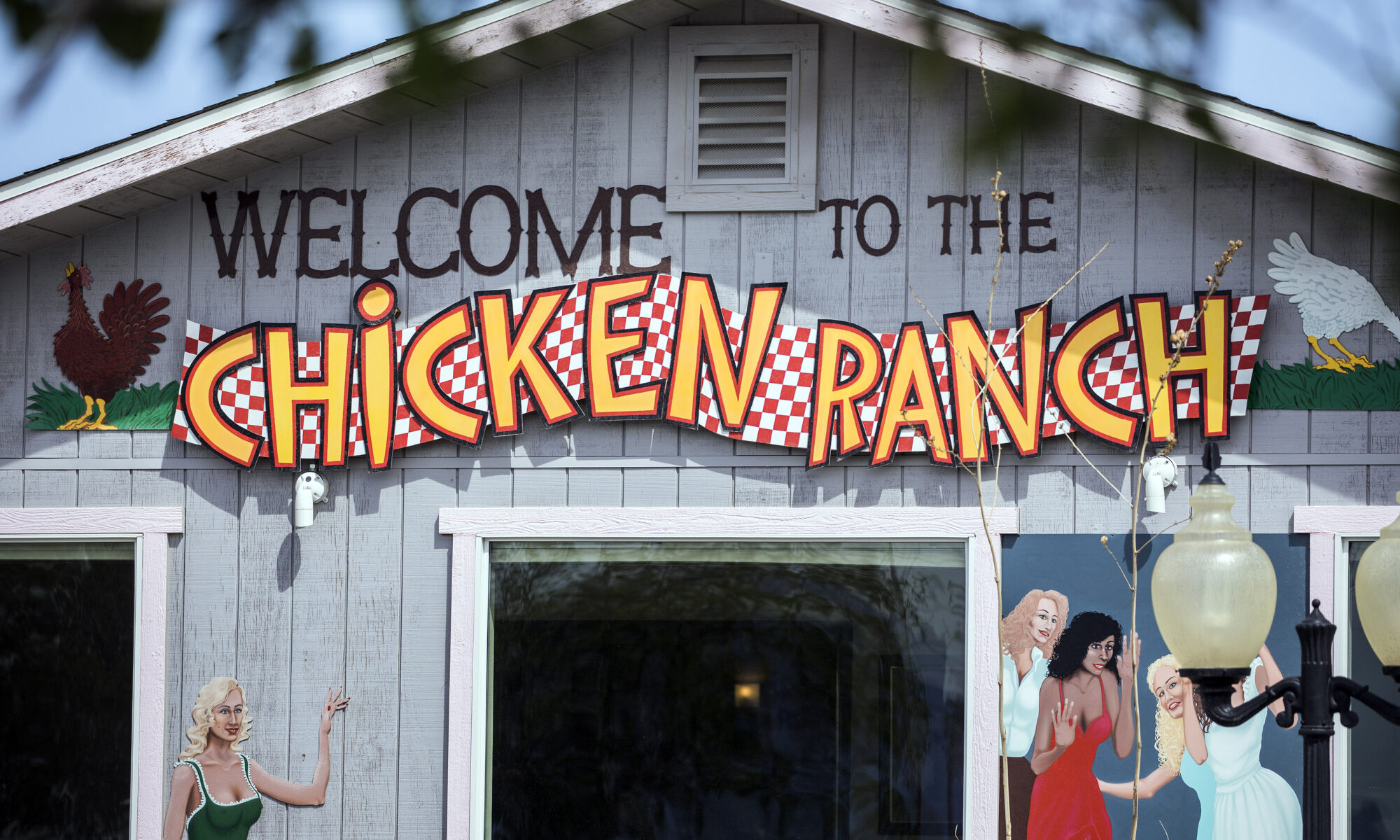The image depicts the front of a barn-style building painted in gray with wooden slats and a distinctive roofline. Dominating the top portion of the building is a large sign reading "Welcome to the Chicken Ranch" in bold yellow letters set against a red and white checkered ribbon-like banner. On the left-hand side of the building, there is a brown rooster, and on the right-hand side, a white chicken. The painting on the barn's facade features various elements: on the lower left, a blonde-haired woman in a green tank top; and on the right, a trio of women, two dressed in blue and one in a red dress with black curly hair, red lipstick, and white painted fingernails. Additionally, a vintage-style black metal light post with globed bulbs is seen in the lower right corner. The entire scene is set under a clear blue sky, adding a picturesque quality to the image.